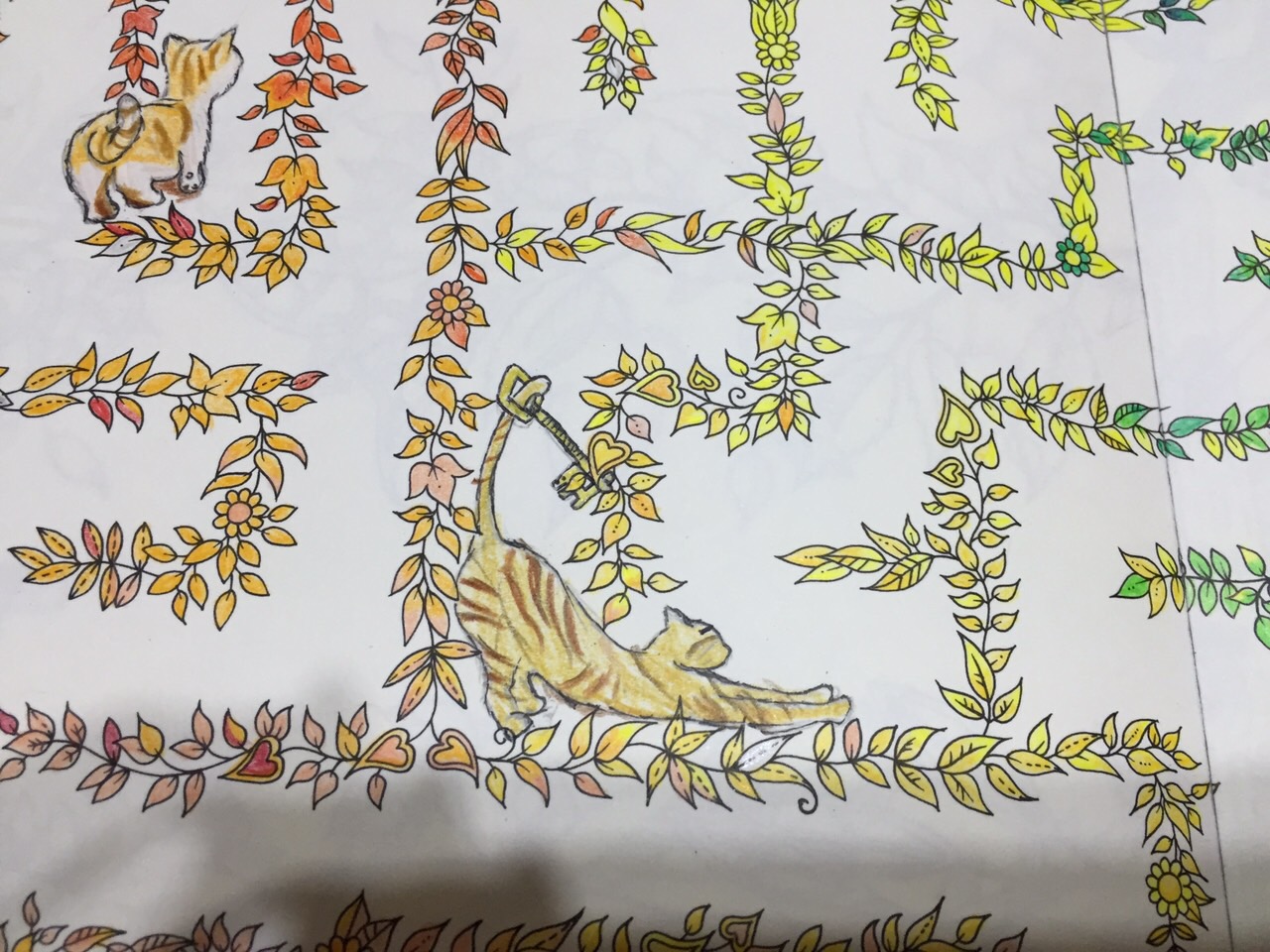The photograph portrays a vibrant piece of artwork set against a pristine white background. The artwork features an intricate pattern of intertwining and crisscrossing strands adorned with leaves. The leaves display a rich spectrum of colors, transitioning from warm autumnal hues on the left, including golden yellows and deep reds, to cooler tones on the right. As the colors shift towards the right, they fade from a vibrant yellow with black edges into darker shades of green.

In the lower section of the artwork, an animated cat is captured in mid-motion. This cat is positioned with its two front paws outstretched forward, leaning down while balancing on its hind legs. In the upper right corner of the image, a second feline figure appears, standing gracefully on all four paws. Both cats are striped, showcasing a combination of dark brown, light brown, and white fur on their chests, adding to the dynamic and lively essence of the artwork.